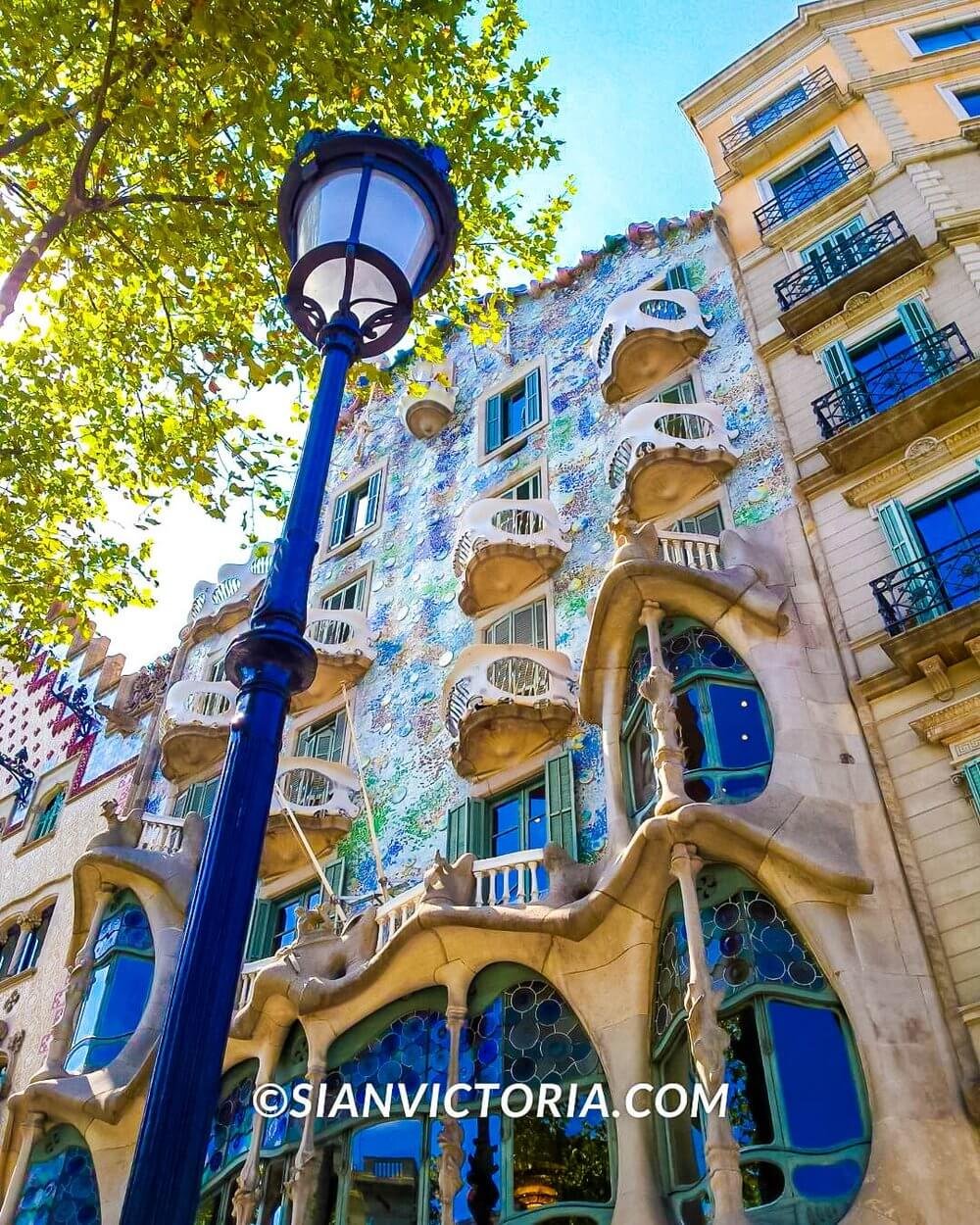This photograph, likely taken for a professional magazine or website, captures the striking side view of a distinctly artistic building, possibly located in Barcelona and inspired by Gaudi's architectural style. The shot is taken midday under a clear blue sky, presenting a six-story structure boasting a facade of brownish stone accented by oval-shaped blue windows, adding to the building's unique and organic aesthetic.

The building's design features a captivating blend of colors: turquoise, green, silver, and crystal-like blue glass pieces that form an eye-catching pattern across the exterior. Some windows are adorned with green shutters and outlined by green windowsills, enhancing the vibrancy of the facade. At the top, a shell-like structure crowns the building, while a black metal railing runs along one side, indicating balconies.

In the foreground, a tall, beautifully painted midnight blue lamppost with a round light fixture stands prominently, complemented by a lush, tall green tree to the right. The photo feels like a postcard image, capturing the essence of the location's architectural beauty and the intricate detailing of the building. The overall composition, from the unusual window shapes to the curved edges, showcases a perfect harmony of colors and forms, making it an architectural masterpiece worthy of feature.

At the bottom of the photograph, in bold white text, the watermark “S-I-A-N-V-I-C-T-O-R-I-A dot com” can be seen, accompanied by a small circle with a 'C' inside, cementing the image's professional grade.